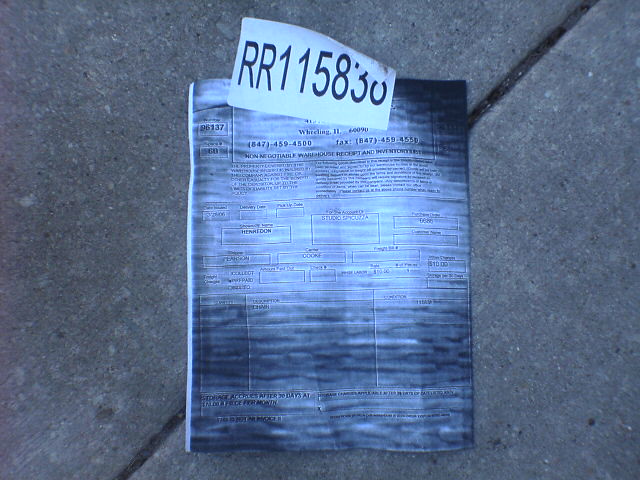This is a high-resolution color image featuring an invoice placed on a dark gray surface. The majority of the invoice is heavily blurred, rendering most of the text unreadable. However, the visible portion at the top of the invoice displays the following information: "Wheeling, Illinois, 60090, 847-459-4500, Fax 847-459-4550, Non-Negotiable Warehouse Receipt and Inventory." A white label bearing the code "RR115838" in black lettering is affixed at the top of the receipt. The right corner of the paper is slightly curling upward. Notably, there are no individuals present in this photograph.